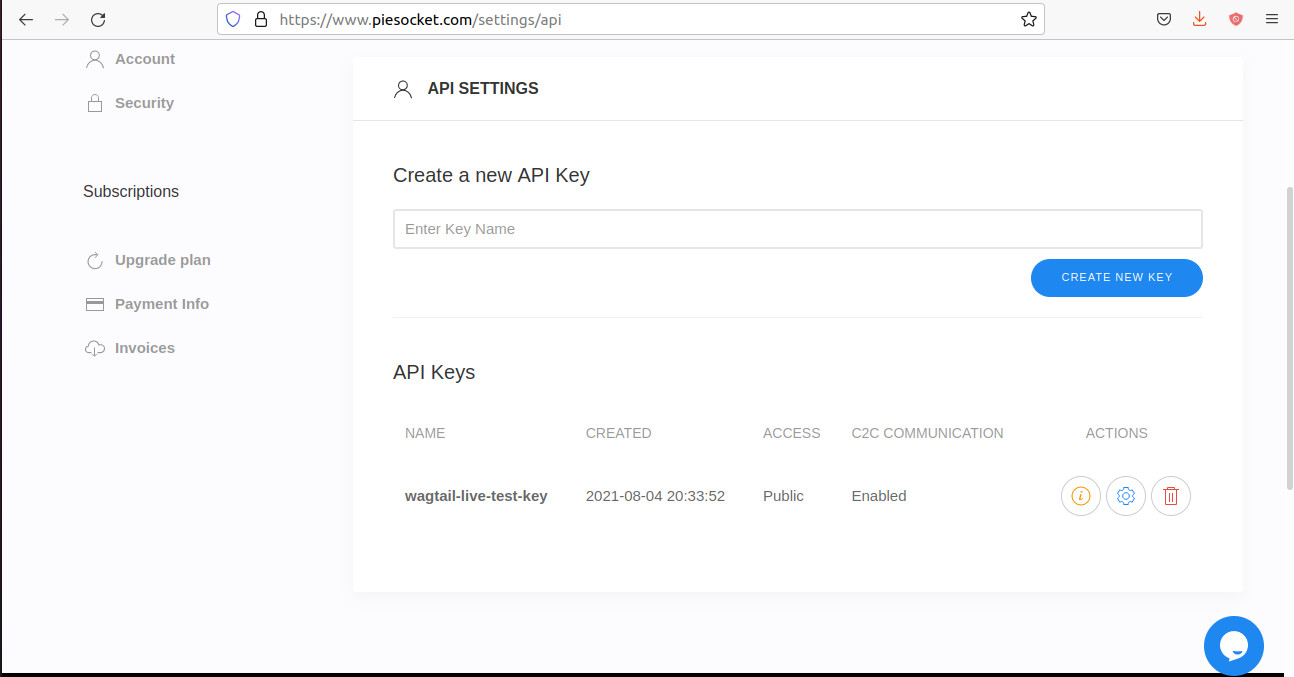This is a detailed screenshot of a web page from www.pysocket.com/settings/API. At the top of the page, the URL is prominently displayed. Along the left-hand side of the screen, a sidebar menu is visible, containing the sections labeled "Account," "Security," "Subscriptions," "Upgrade Plan," "Payment Info," and "Invoices."

Dominating the center of the image is the header "API SETTINGS," rendered in bold, uppercase letters. Below this header, there is a prompt that reads "Create a New API Key," followed by a rectangular input field designated for entering the key name. Adjacent to this input field, on its right side, there is a prominent blue oval button labeled "Create New Key." 

Further down, the page displays the section titled "API Keys," where columns for "Name," "Created," and "Access" (specifically "C2C Communication") are visible next to a column for "Actions."